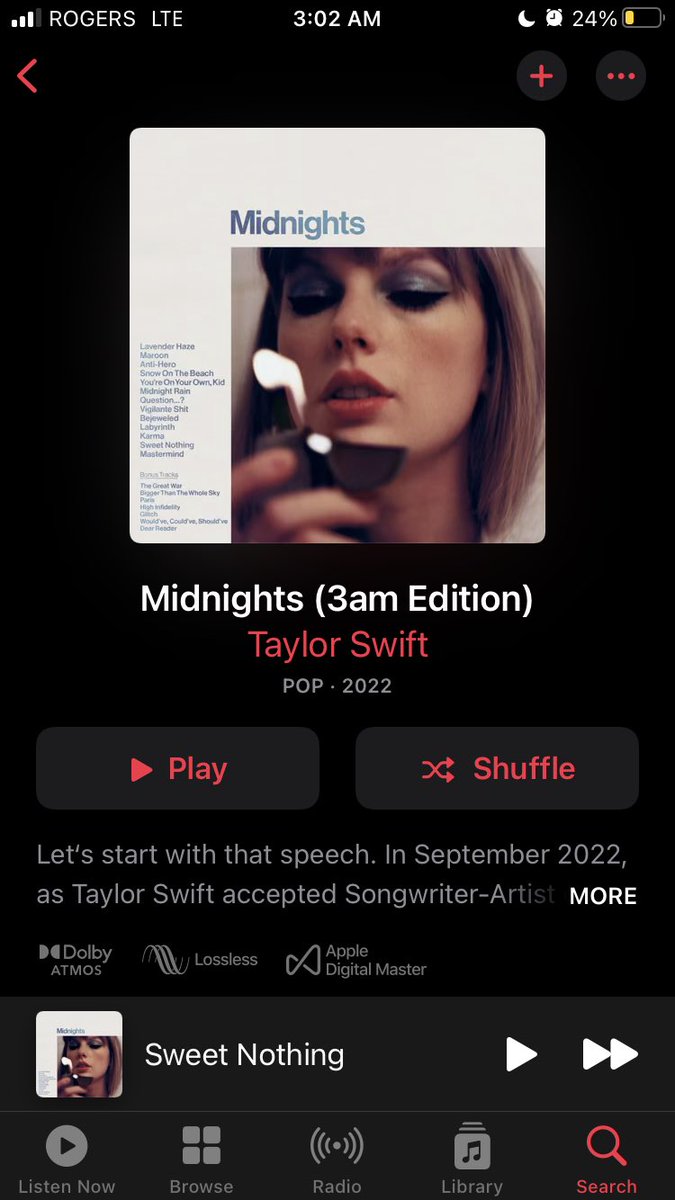In this screenshot of a cellular device, the status bar at the top captures several details: the battery is at 24%, noted by a small yellow block indicating low battery; an alarm is set, denoted by an alarm clock icon; and a crescent moon icon on the left side of the time suggests Do Not Disturb mode is on. It is 3:02 AM, and the network status shows "Rogers LTE" with three out of four signal bars.

The screen prominently displays an album by Taylor Swift titled "Midnight's (3 AM Edition)." Below the album title, it reads "Pop 2022, Taylor Swift," where "Taylor Swift" is highlighted in red text, along with the play and shuffle buttons. A snippet of text follows, starting with "Let's start with that speech in September 2022," and indicating Taylor Swift's acceptance of an unspecified award, before trailing off.

Further down, a larger white text indicates "more." Below this, a rectangular banner features the track "Sweet Nothing" and showcases the album cover again. The cover has a white background with "Midnight's" written in faded blue. Taylor Swift appears on the cover with blue faded eyeshadow, red lipstick, and subtle bangs, looking down at a lighter in her right hand. Finally, at the bottom of the screen, there are navigation icons for "Listen Now," "Browse," "Radio," "Library," and "Search."